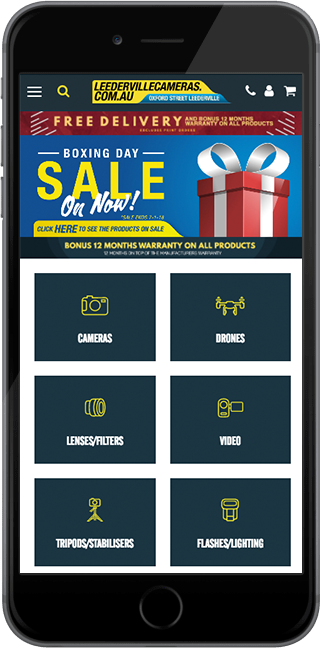Here's a cleaned-up and detailed caption for the image:

---

**Image Description:**

This image is a mock-up of a webpage for "leadervillecameras.com.au," displaying on an older black iPhone with signature curved lines. The iPhone is characterized by a black area at the top and bottom and a black home button at the bottom center. The metal frame of the device is visible, featuring three buttons on the left side. The entire device is set against a clean white background.

On the webpage, a red header announces "Free Delivery" in bold text. Below this header, there is an eye-catching advertisement promoting a Boxing Day sale, featuring a 3D gift box wrapped with a white bow. Accompanying this ad, white and yellow text invites users to "Click here to see products on sale" and highlights a "Bonus 12 months warranty on all products."

Directly beneath the ad, there are six menu options laid out in two columns and three rows, each set on a blue field. The menu icons are yellow with white text descriptions:

1. **Top Left:** An icon of a camera with the label "Cameras."
2. **Top Right:** An image of a drone labeled "DRONES" in a thin, all-capital font.
3. **Middle Left:** A camera lens icon next to the text "Lenses / Filters."
4. **Middle Right:** A video camera with a fold-out screen labeled "Video."
5. **Bottom Left:** A tripod with a mounted camera, described as "Tripod / Stabilizers."
6. **Bottom Right:** A simple flash icon labeled "Flashes / Lighting."

Additionally, the top navigation bar of the webpage features icons for a search function, a call button, a user profile, and a shopping cart. 

---

This detailed caption provides a thorough description of the webpage layout and contents, giving a clear picture of the scene depicted.